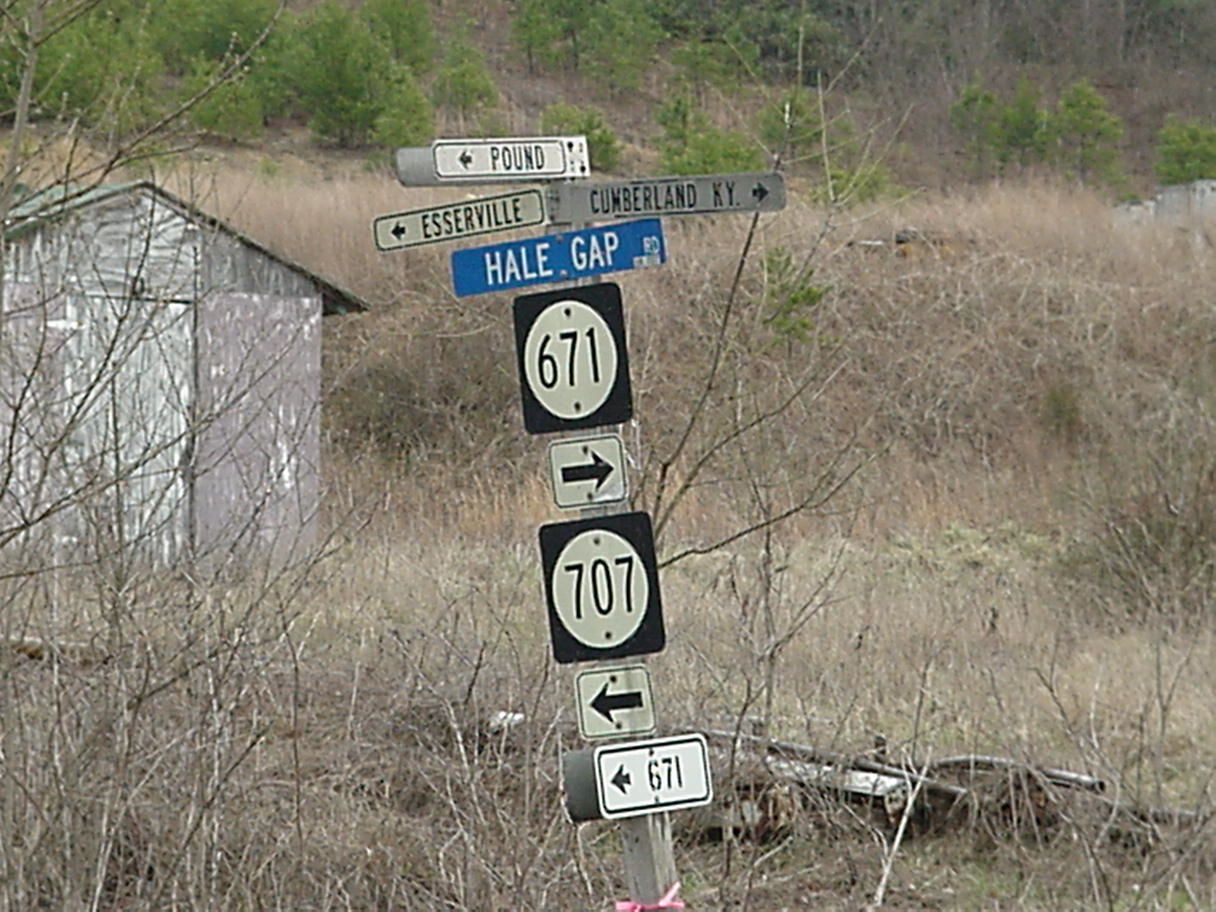This photograph captures a slightly tipped-over road sign situated in a wooded area teeming with bare branches and trees that stretch into the skyline. The left side of the frame reveals a slightly rundown shack, light brown in color with white weathering and a blackened roof, partially hidden among the trees. Behind the road sign, some scattered fallen wooden objects can be seen. The road sign itself is adorned with multiple directional indicators: 

- At the top, three names are listed: Pound, Estherville, and Cumberland, Kentucky.
- Below this, a blue sign reads "Hale Gap."
- A black sign with a white circle displays the number 671 and an arrow pointing to the right.
- Another similar sign indicates 707 with an arrow pointing to the left.
- Finally, a rectangular sign at the bottom reads 671 with an arrow also pointing to the left.

The scene is an intriguing blend of natural and man-made elements, offering a glimpse into a rustic and slightly dilapidated rural environment.